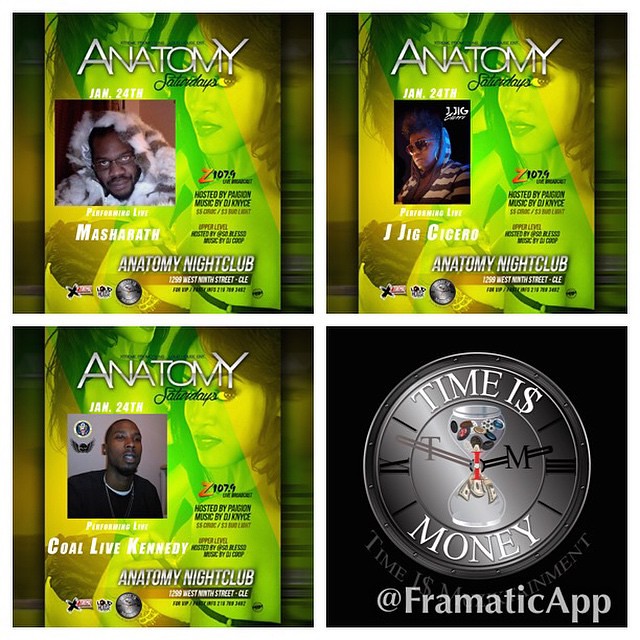This is a detailed promotional collage for Anatomy Nightclub in Cleveland, Ohio, featuring four distinct images. The top left quadrant is an advertisement for "Anatomy Saturdays," showcasing a neon green and yellow background with a woman looking straight ahead. Directly to the right, another ad highlights the same "Anatomy Saturdays," with a black woman wearing a black and white striped hoodie. Both ads list event details, including performances by Masha Rath, J. Jig Cicero, and Cole Live Kennedy on January 24th.

In the bottom left quadrant, another flyer features a black male looking to the side, dressed in a black t-shirt and necklace, overlayed on the same neon background. This quadrant again emphasizes the Saturday night event and lists the nightclub's address as 1258 West 9th Street, CLE. The promotional text mentions hosting by Pageon Music, DJ Nice (Knyce), and sponsored specials like $5 Ciroc and $3 Bud Light.

The bottom right quadrant is a distinct image of a clock with an hourglass in the center, framed by the phrase "Time is Money." This serves as a logo for the promotional campaign, tied to the social media handle @FromaticApp.

Overall, this well-rounded advertisement captures the vibrant atmosphere of Anatomy Nightclub's Saturday events, highlighting both the performers and immersive party experience, underscored by the slogan, "Time is Money."